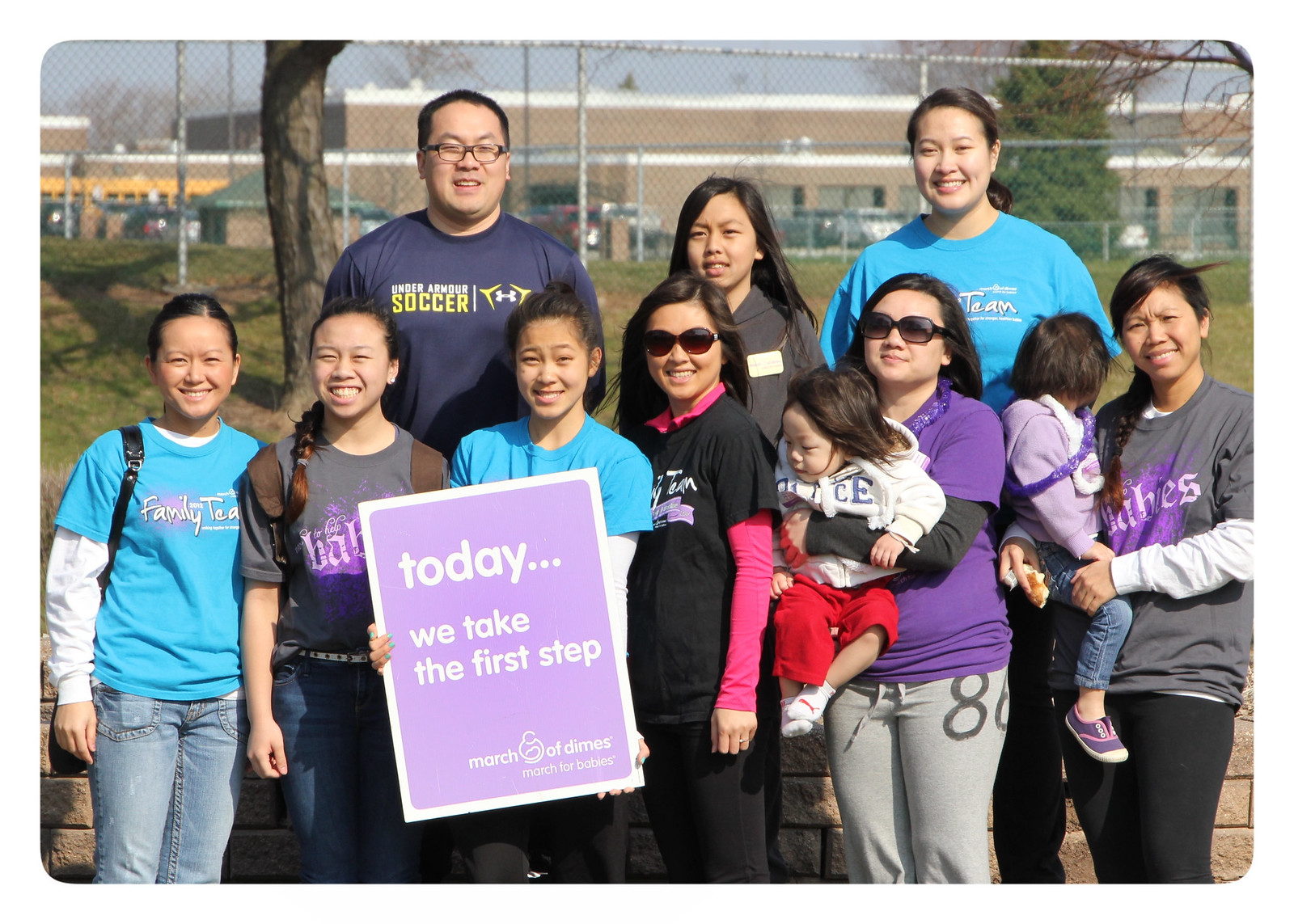In this vibrant photo, a group of eleven people, primarily of Asian descent, are gathered in a park, posing for the camera against a backdrop of trees, grass, and a building with a chain-link fence in the distance, suggesting a school setting. The group is composed of men, women, children, and toddlers, all standing in two rows and dressed in casual attire, including blue, purple, and black t-shirts with long sleeves underneath, indicative of a sunny yet slightly cool day. Prominently, a teenage girl in a blue shirt stands at the center, holding a purple sign with white text that reads, "Today we take the first step," associated with a March of Dimes event. To the right, a mother and another girl each hold a young child, adding a familial touch. Two women and a man are visible in the background, with the man wearing a shirt that references soccer. Many in the group are smiling, some sporting sunglasses, enjoying the bright day as they unite for this cause.